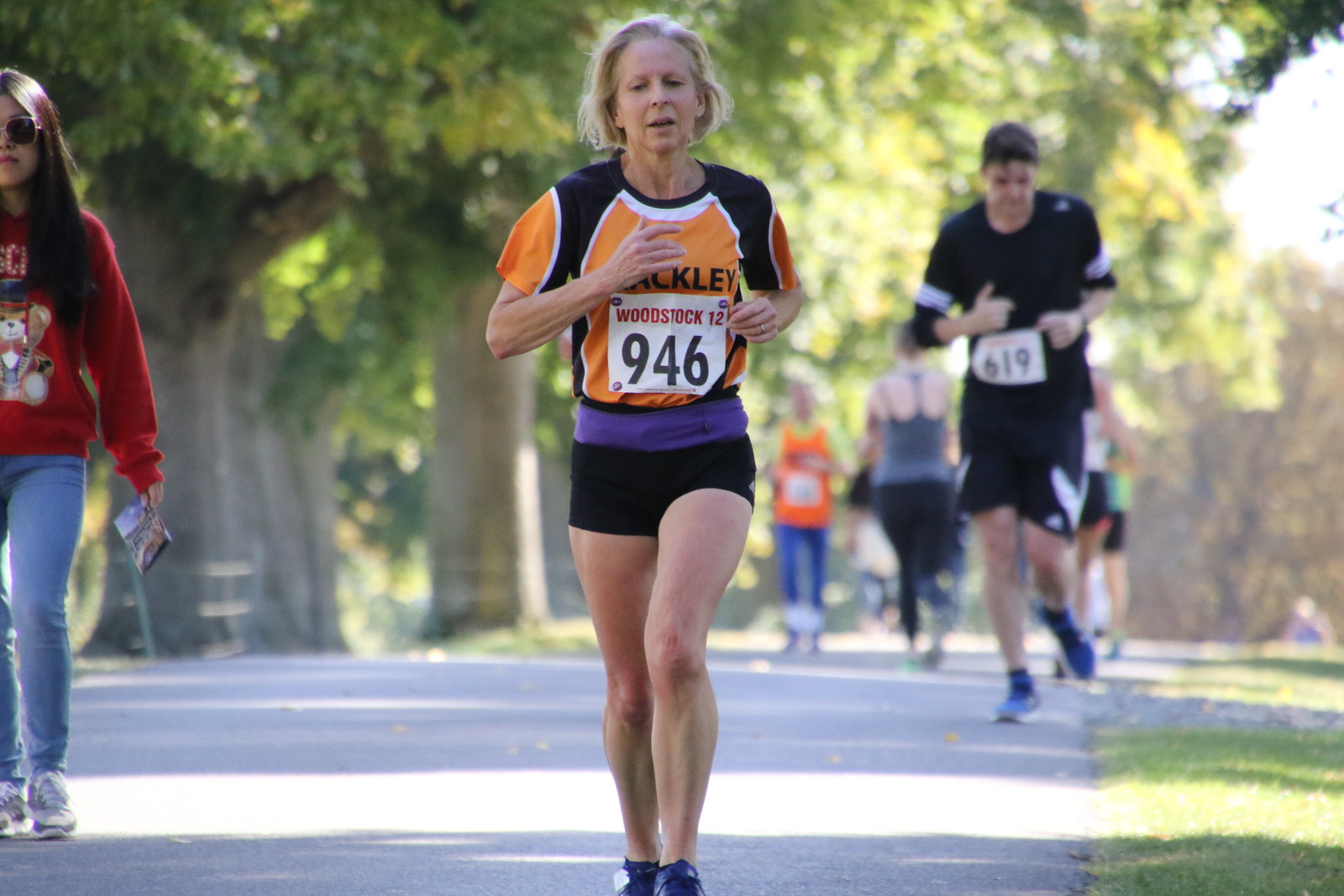In this vibrant photograph of a marathon, a bustling scene unfolds on a flat, light gray asphalt path flanked by grassy fields. On the left side of the path, thick-trunked trees with lush, green leaves add a touch of nature's beauty to the background. The focal point of the image is a determined woman mid-stride at the center, clad in short black shorts and an eye-catching orange t-shirt with black shoulders, white stripes, and a white neckline. A purple sash adds a dash of color. Pinned to her jersey is a paper reading "Woodstock 12-946." Just behind her, another runner, dressed entirely in black and wearing a bib with the number "619," strides forward. To the left side of the road, a woman in jeans and a long-sleeved red shirt walks along, providing a contrast to the runners. In this moment, the energy and diversity of participants in the marathon are vividly captured.